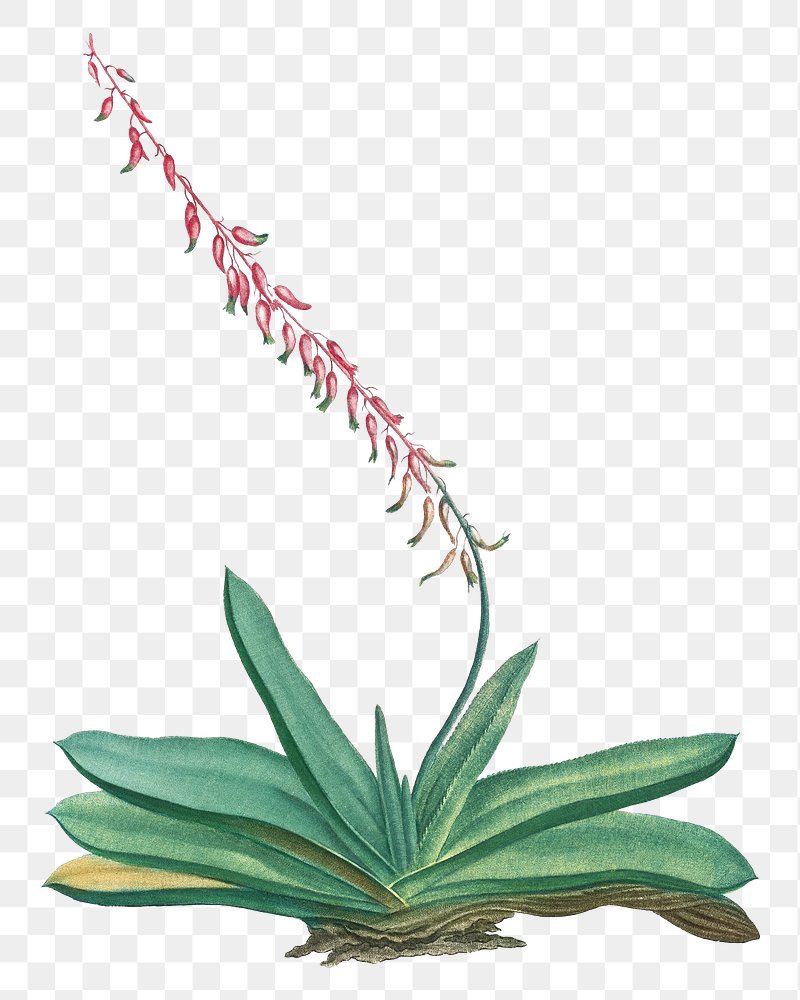Against a gray and white checkered background, indicative of a transparent layer typically seen in image editing software like Photoshop, there is a detailed illustration of a plant. At the bottom center, the plant has a base composed of brownish stems with several wide and elongated green leaves, resembling an aloe vera plant. The outermost leaves are larger and spread outward, while the leaves closer to the center get progressively smaller. Notably, the bottom left leaf has a yellow tip, contrasting with the predominantly green and brown hues of the other leaves.

From the center of the plant, a thin green stem extends upwards, diagonally reaching towards the top left corner of the image. Attached to this stem are several small, tadpole-shaped buds or petals that are pinkish-red in color, resembling tiny chili peppers or young flower buds. The stem and its buds add an element of dynamic growth to the image, suggesting potential blooming. The detailed illustration captures the intricate variations in leaf size and coloration, coupled with the delicate, colorful budding along the slender stem, set against the semi-transparent checkered backdrop.